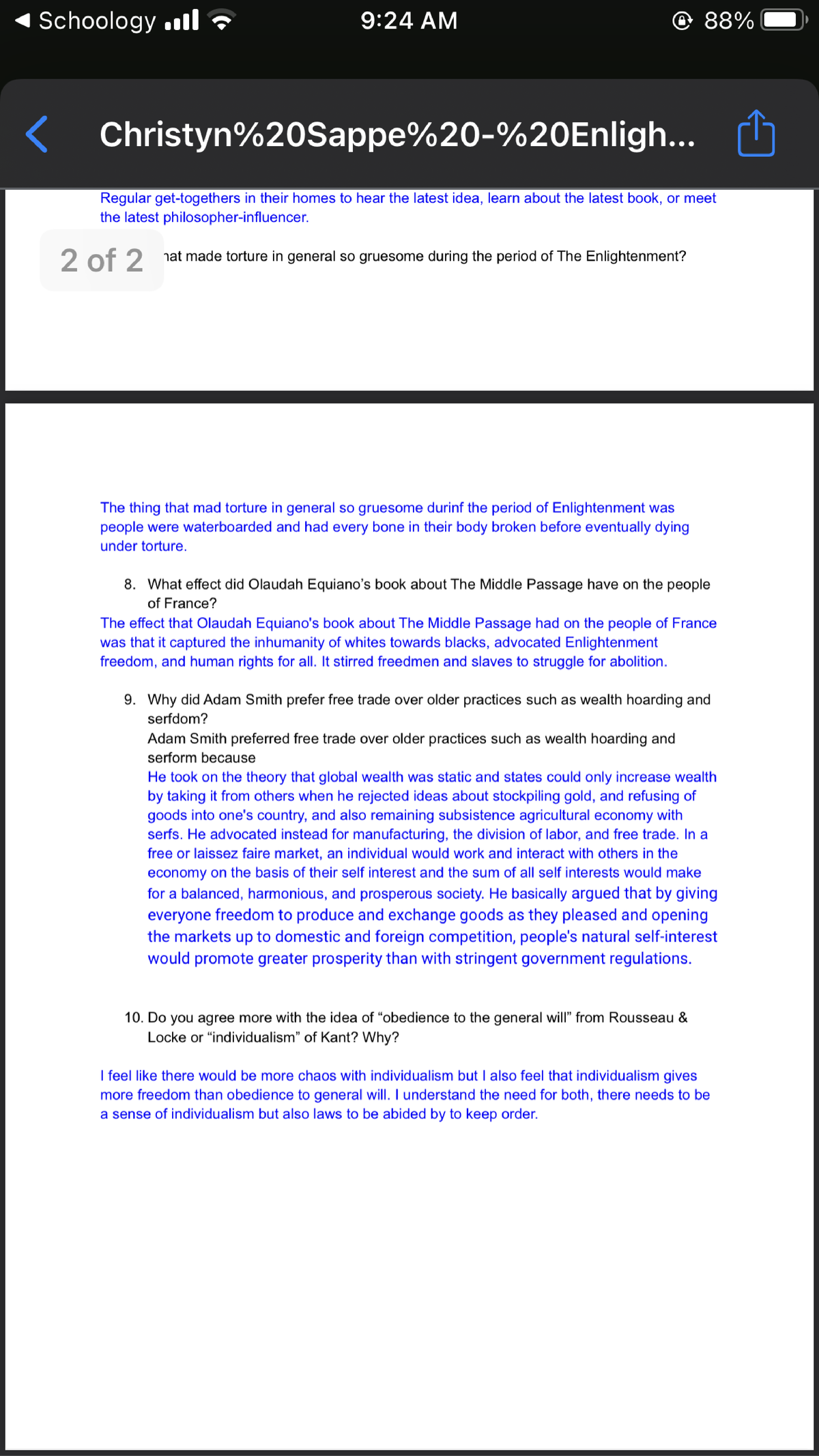This screenshot from Schoology features a predominantly white background. At the top, a black rectangle spans from left to right, displaying the word "Schoology" in white text alongside icons indicating signal strength and Wi-Fi connectivity. Centrally located, "9:24 AM" is presented in white text, accompanied by "88%" and a battery indicator to the right.

Below this header, a charcoal gray rectangle appears with white text reading, "Christian 20% SAP % 20 - % 20 English." The subsequent section of the interface showcases a white background with blue and black text. The blue text begins with "regular get-togethers in their homes to hear the latest idea, learn about the latest book, or meet the latest philosopher, influencer." This text fragment leads into a discussion about the period of the Enlightenment, stating, "The thing that made torture in general so gruesome during the period of Enlightenment was people were waterboarded and had every bone in their body broken before eventually dying under torture."

In black text, item number eight poses the question, "What effect did Oluda Equiano's book about the Middle Passage have on the people of France?" The blue text response follows: "The effect that Oluda Equiano's book about the Middle Passage had on the people of France was that it captured the inhumanity of whites towards blacks, advocated Enlightenment freedom, and human rights for all. It stirred freedom and slaves to struggle for abolition."

The next question, number nine, asks, "Why did Adam Smith prefer free trade over older practices such as wealth hoarding and serfdom?" The extensive blue text reply explains: "Adam Smith preferred free trade over older practices such as wealth hoarding and serfdom because he took on the theory that global wealth was static and states could only increase wealth by taking it from others. He rejected ideas about stockpiling gold and refusing goods into one's country, as well as remaining subsistence agricultural with serfs. He advocated instead for manufacturing, the division of labor, and free trade in a free or laissez-faire market where individuals could work and interact based on their self-interest. The sum of all self-interest would create a balanced, harmonious, and prosperous society. He argued that by giving everyone freedom to produce and exchange goods and opening markets to domestic and foreign competition, people's natural self-interest would promote greater prosperity than stringent government regulations."

Finally, question number ten in black text asks, "Do you agree more with the idea of obedience to the general will from Rousseau and Locke or individualism from Kant? Why?" The response reads: "I feel like there would be more chaos with individualism but also feel that individualism gives more freedom than obedience and general will. I understand the need for both. There needs to be a sense of individualism but also laws need to be abided by to keep order."